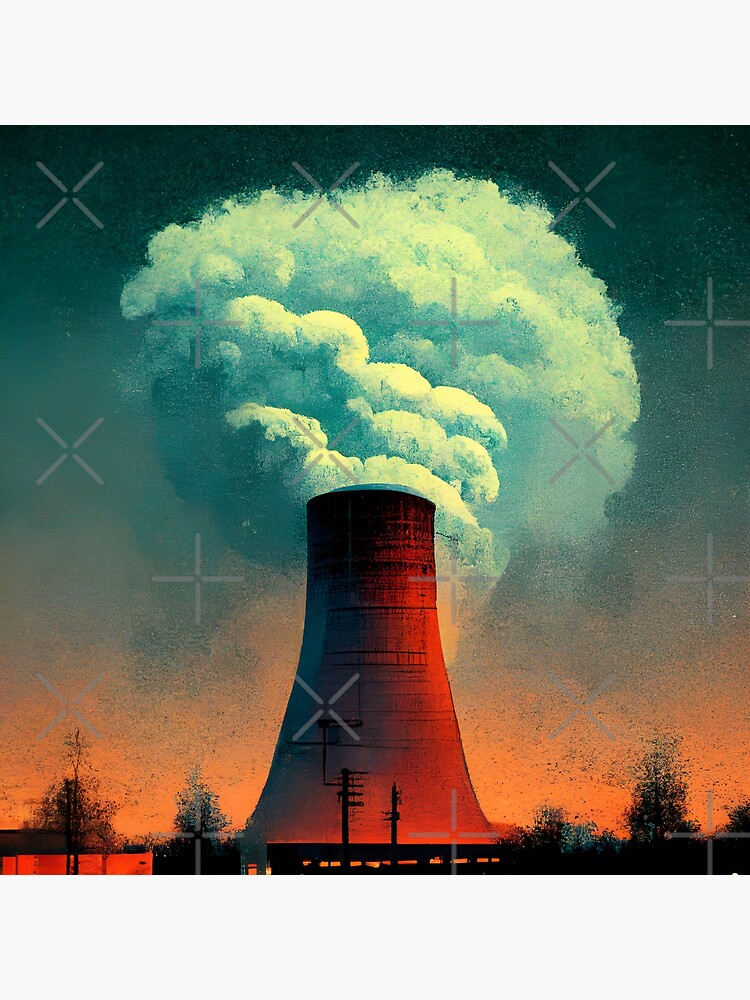This illustration of a cooling tower at a nuclear power plant presents a striking visual with distinct color contrasts and detailed elements. The right-hand side of the tower is bathed in a red hue from an off-frame light source, while the left side remains shrouded in shadow, appearing black. The tower's enormous structure is emphasized by a towering plume of steam or smoke that billows out from its top, with white highlights and blue shadows. The horizon behind the tower glows orange, suggesting a sunrise or sunset, against a sky that transitions to blue. The base of the tower features two telephone or utility poles, and there are small trees flanking both sides—each about a fifth the size of the tower. Additionally, the image contains watermarked pluses and X marks for copyright protection. The scene includes notable details like potential railway tracks or dark lines near the foreground, adding depth and complexity to this high-quality print or painting.